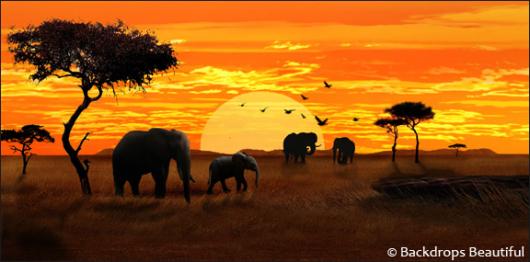The image captures a breathtaking scene of elephants on a grassy savanna during sunset. In the foreground, an adult elephant and a baby elephant are seen strolling towards the right, with two larger elephants framed by trees in the background. The sky is a vibrant display of deep orange and yellow hues, creating a striking array of colors as the sun dips towards the horizon. Silhouettes of birds are seen flying near the radiant sun, adding to the image's serene beauty. Darker-colored trees punctuate the scene, their silhouettes enhancing the texture of the imagery. The composition is completed with the text "© backdrops beautiful" positioned in the bottom right corner, adding a note of authenticity to this mesmerizing snapshot of nature.